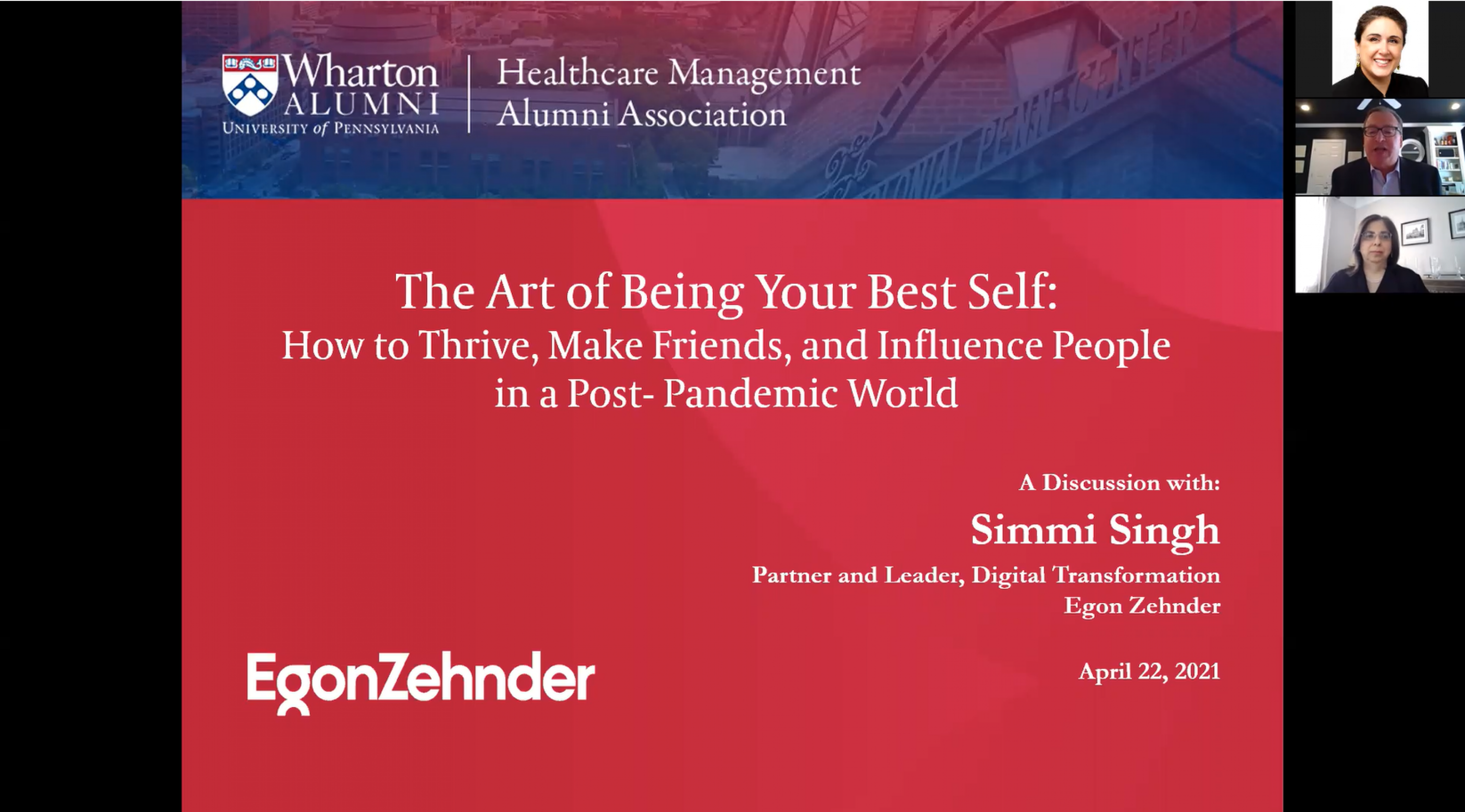This screenshot captures a virtual meeting featuring a presentation at the center of the screen. On the right side, three participants are displayed: a static photo of one individual at the top, and live video feeds of a man and a woman beneath. The presentation's slide, dominated by a red background with white text, is titled "The Art of Being Your Best Self: How to Thrive, Make Friends, and Influence People in a Post-Pandemic World." It is presented by the Wharton Alumni, University of Pennsylvania Healthcare Management Alumni Association. The session is led by Simi Singh, a partner and leader in Digital Transformation at Egon Zender, and took place on April 22, 2021. The upper section of the slide features a blue overlay with the University of Pennsylvania's logo and an image of the college campus, including its iconic wrought iron signage.